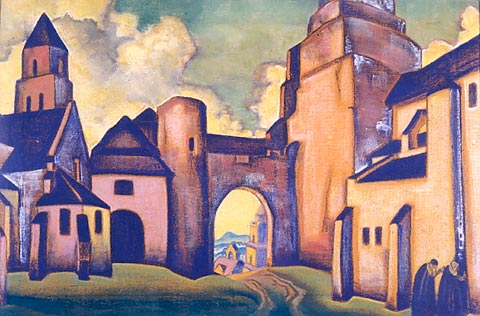This artwork, a whimsical painting or drawing, depicts a large, bucolic estate or village with an adobe-like architectural style. The buildings, rendered in shades of beige, pink, and brown to add depth and texture, form a cohesive yet varied skyline. Starting from the left, a tall, cylindrical tower with a narrow vertical opening stands prominently. Adjacent to it is a classic-shaped structure that features a domed opening, hinting at castle-like inspiration. Moving to the right, there's a smaller tower resembling a barn opening and an archway that U-shapes into an open path, leading the viewer's eye towards additional buildings in the background. A significant segment on the far right, seemingly larger than the left tower, perhaps alludes to a church. This inference is bolstered by the presence of two robed figures, likely monks or priests, situated in the lower right corner. The foreground is dotted with green grass, contrasting with the blue sky above, filled with thick, billowy clouds accented with hints of yellow. The overall palette includes browns, whites, blacks, greens, grays, blues, tans, and touches of pink and yellow, making the scene lively and texturally rich.